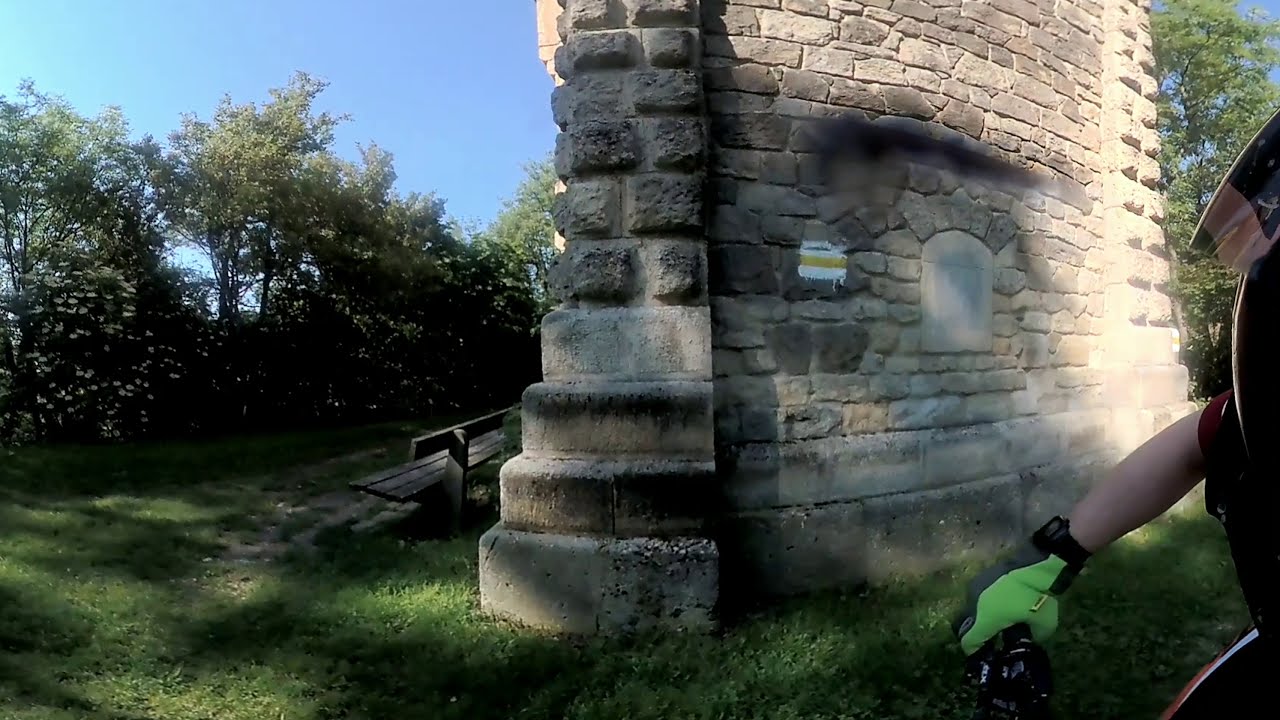The outdoor scene captured in the image features a tall, cobblestone brick wall with varying sizes and shapes of bricks, reminiscent of a Renaissance castle. The wall, slightly distorted in the photo, includes an arched window filled in with concrete in the center, and to its left, a rectangular spot marked with white paint and a yellow stripe. On the left side of the wall is a wooden bench. Further to the left, towards the bottom center of the image, a wooden ramp is visible, suggesting possible access to the structure. Dominating the right side of the image, a biker is partially captured, showing only the right shoulder and arm adorned with a short sleeve shirt, a black watch, and a distinctive green glove gripping the bike's handlebars, with a thigh in black leggings visible below. The background and foreground are lush with green grass and trees under a clear blue sky, reinforcing the outdoor setting. The image is a color, landscape-oriented panoramic photograph that seamlessly blends two views of the same subject, providing a realistic depiction of the scene.